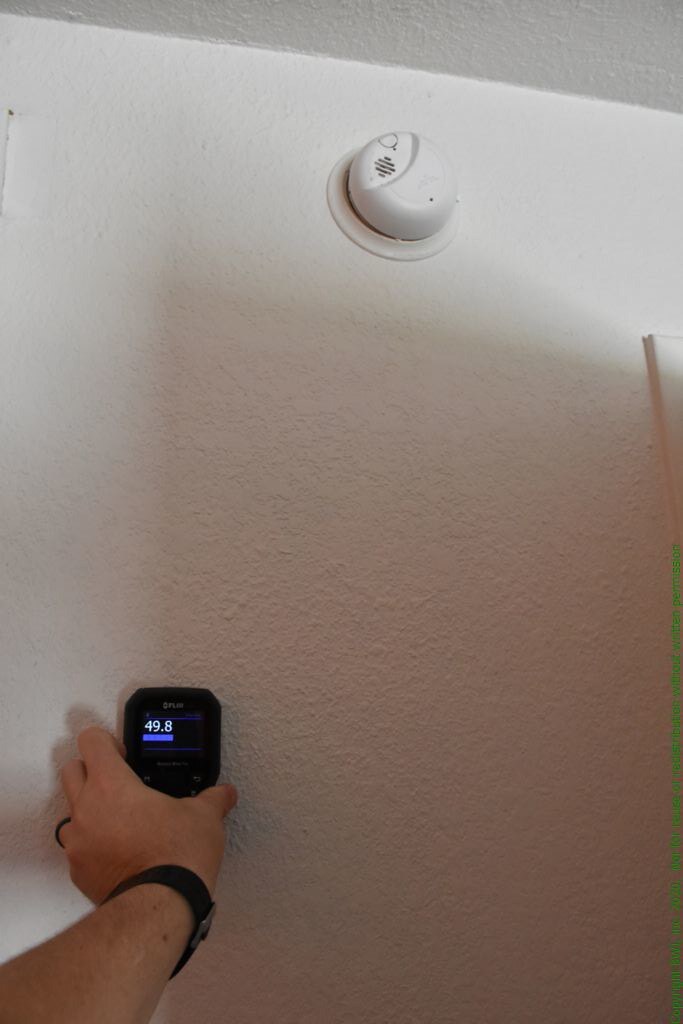The image depicts a transition from a white wall and white ceiling to a pinkish-brown gradient. At the top of the wall, there's a white fire detector featuring subtle pink shadows and black detailing, including a dot on the right side. A hand, adorned with a black wrist accessory and a black ring, holds a black device displaying the number "49.8" on its screen, accompanied by a purple bar underneath. The hand's shadow is cast onto the wall, blending into the pinkish-brown hue. Along the right-hand side of the image, about a quarter way down, there is a thin black line and two darker gray lines that fade into the background. Additionally, a fragmented green stripe is visible on the right side, complementing the pinkish-brown color scheme.